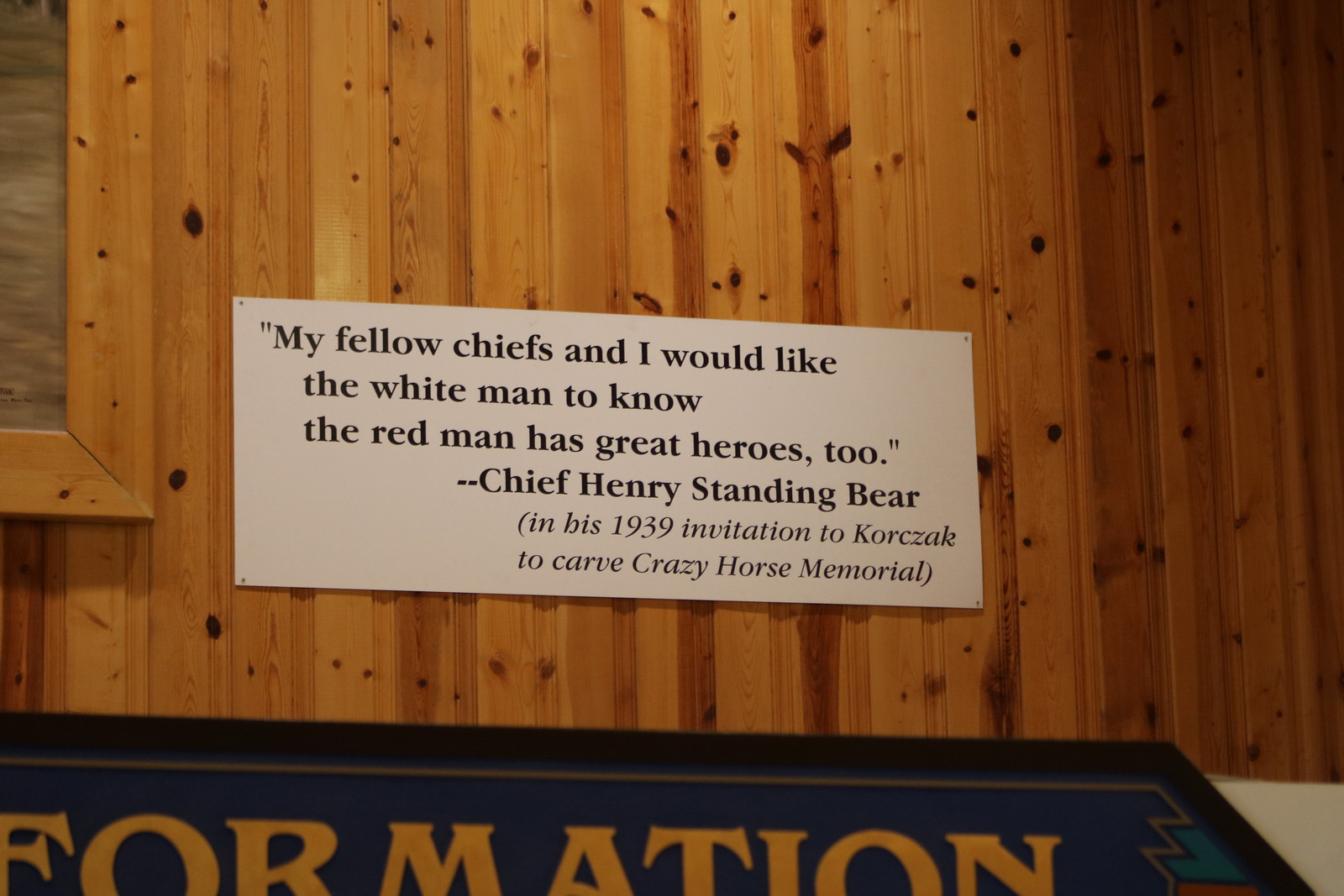The image shows a white sign with black text mounted on a vertical pinewood wall. The sign reads: "My fellow chiefs and I would like the white man to know the red man has great heroes too. Chief Henry Standing Bear in his 1939 invitation to Korczak to carve the Crazy Horse Memorial." To the left of the sign, there is a trim-like structure resembling the outline of a window or cupboard. At the bottom of the image, partially obscured, is another blue sign with black border and frame, showing the word "formation," likely part of the word "information." The wooden wall has visible grain and markings, and above the white sign, the corner of a picture frame can be seen.